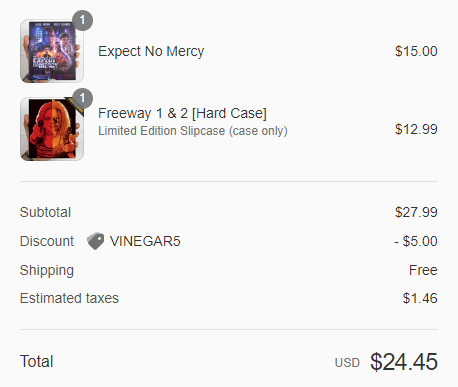This screenshot showcases a checkout page for a purchase of media items. The first item listed is titled "Expect No Mercy," which appears to be either an album or a movie, displayed with its cover art predominantly featuring blue and red colors. It's priced at $15.00. The second item is "Freeway 1 and 2 Hard Case, Limited Edition, Slipcase Case Only," priced at $12.99, with its cover art primarily in various shades of red.

Below the item listings, the subtotal is shown as $27.99. The page also indicates a discount code "VINEGAR5" which deducts $5.00 from the subtotal. Shipping is noted as free, and the estimated taxes are calculated at $1.46. The total amount due is displayed as $24.45 USD at the bottom of the page.